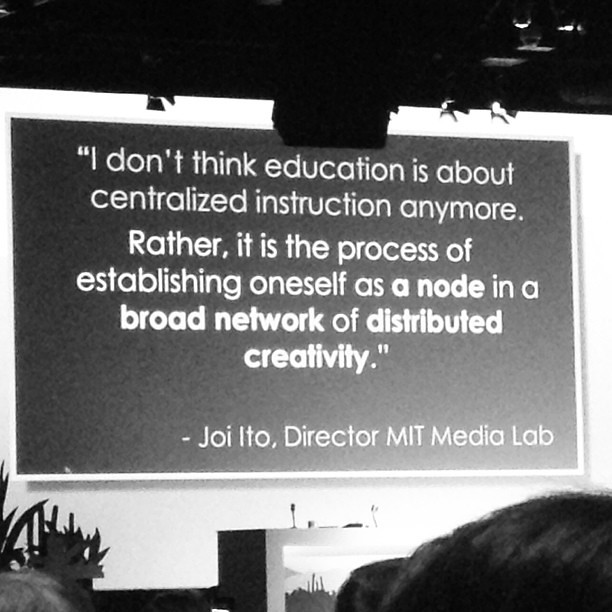A black and white photograph captures a moment in a conference hall, where an audience is engaged in a presentation. The image shows the backs of attendees' heads at the bottom, directing their attention towards a podium situated centrally on a stage. Above the podium, a large projection screen displays a quote that reads, "I don't think education is about centralized instruction anymore. Rather, it's a process of establishing oneself as a node in a broad network of distributed creativity." This profound statement is attributed to Joi Ito, Director of the MIT Media Lab. The ceiling of the auditorium is visible, illuminated by an array of lights that subtly enhance the atmosphere of the gathering. The overall ambiance is one of intellectual engagement and discourse.